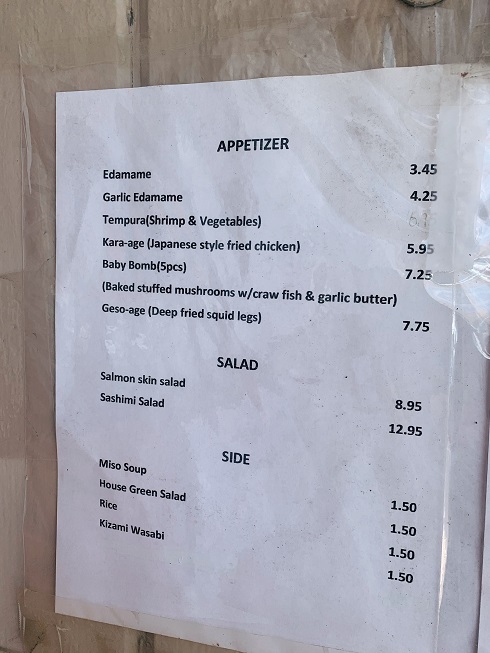The image features a printed menu displayed prominently on a brown wooden wall, secured with visible tape on the right side. The menu itself is a white piece of printer paper with black text, structured simply and clearly. At the top in all capital letters is the header "APPETIZER," under which a list of appetizers is presented: edamame, garlic edamame, tempura, karaage (Japanese fried chicken), baby bomb, baked stuffed mushrooms, and gizoage (deep-fried squid legs). Below the appetizers section, the menu transitions to "SALAD," also in all caps, listing two options: salmon skin salad and sashimi salad. Further down, the word "SIDE" appears in bold uppercase letters, detailing side dishes such as miso soup, house green salad, rice, and kazami wasabi. All listed items have their corresponding prices neatly aligned to the right of their names.